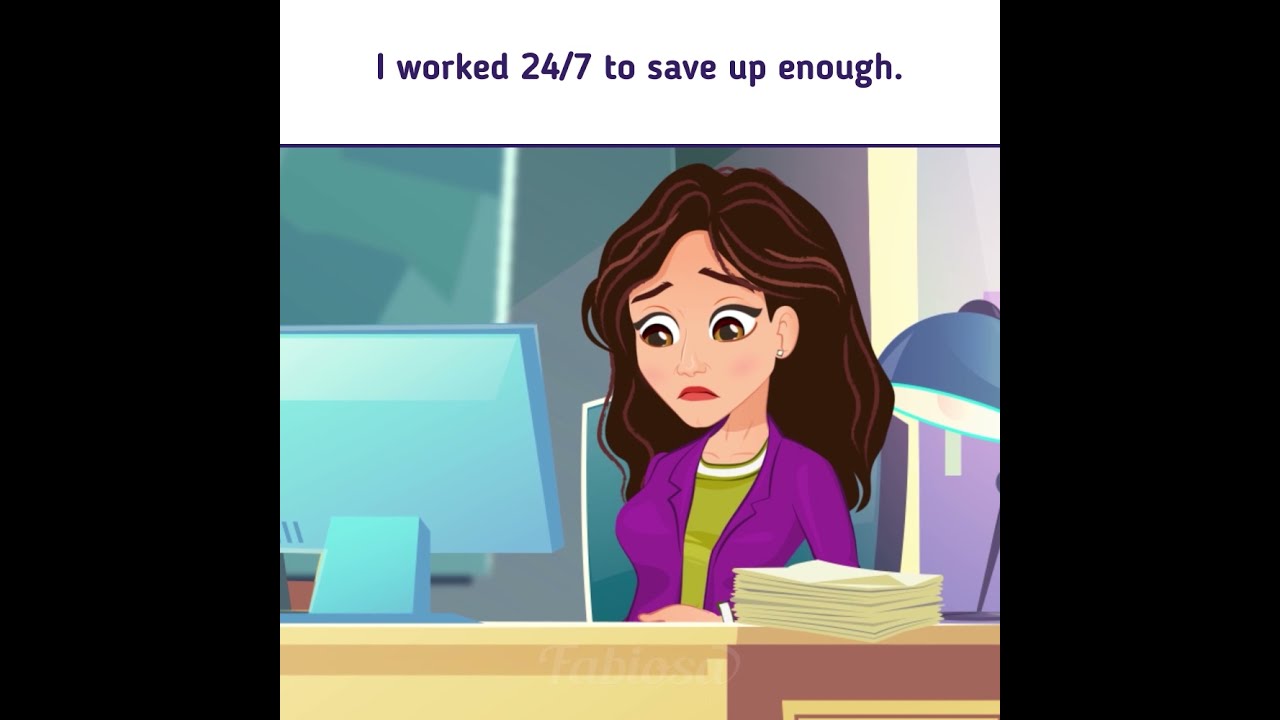The image is a wide rectangular cartoon with black bars on the left and right sides. In the middle, a woman is seated at a wooden desk, looking down at her computer screen with a concerned expression, as indicated by her raised eyebrows. She has big brown eyes, light brown hair with streaks, and is wearing a purple jacket over a green shirt with a white scooped collar. Her lips are adorned with red lipstick, and she has an earring on her left ear. To her right is a stack of yellow papers, and behind her to the right is a blue lamp, shining straight down, signaling that it's on. The woman's desk hosts a computer with a light blue back and a rectangular arm supporting it. Above her, a white bar with dark purple text reads, "I worked 24-7 to save up enough."